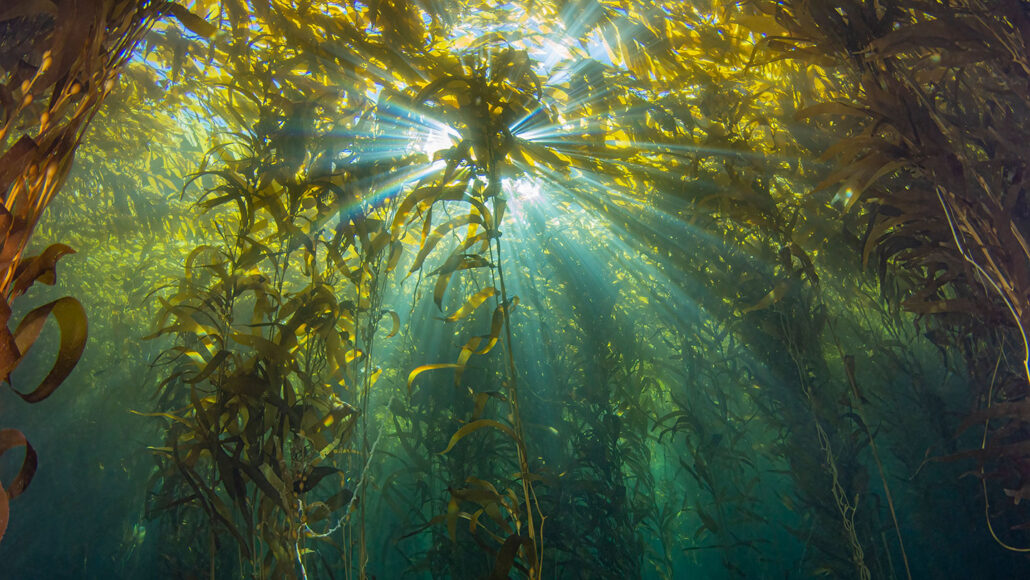This underwater photograph, taken during the day, captures an ethereal scene of a vibrant underwater ecosystem, bathed in sunlight streaming through the water. Looking up from the seabed, the dense canopy of kelp and seaweed forms a mesmerizing forest-like ceiling that diffuses the sunlight into beautiful rays. The sunlight filters down through the clear water, creating a spectrum of turquoise and green hues that lend the scene a haunting yet captivating ambiance. Various underwater plants, predominantly in greenish-yellow tones, dominate the image. Notably, an orange plant anchors the left side of the frame, while a striking yellow plant stands out on the right. The sunlight bathes a group of yellow plants, accentuating their colors and making them glow against the clear backdrop. The overall effect is a stunning interplay of light and color, evoking a sense of serene submersion and a hint of the eerie depth of the ocean.